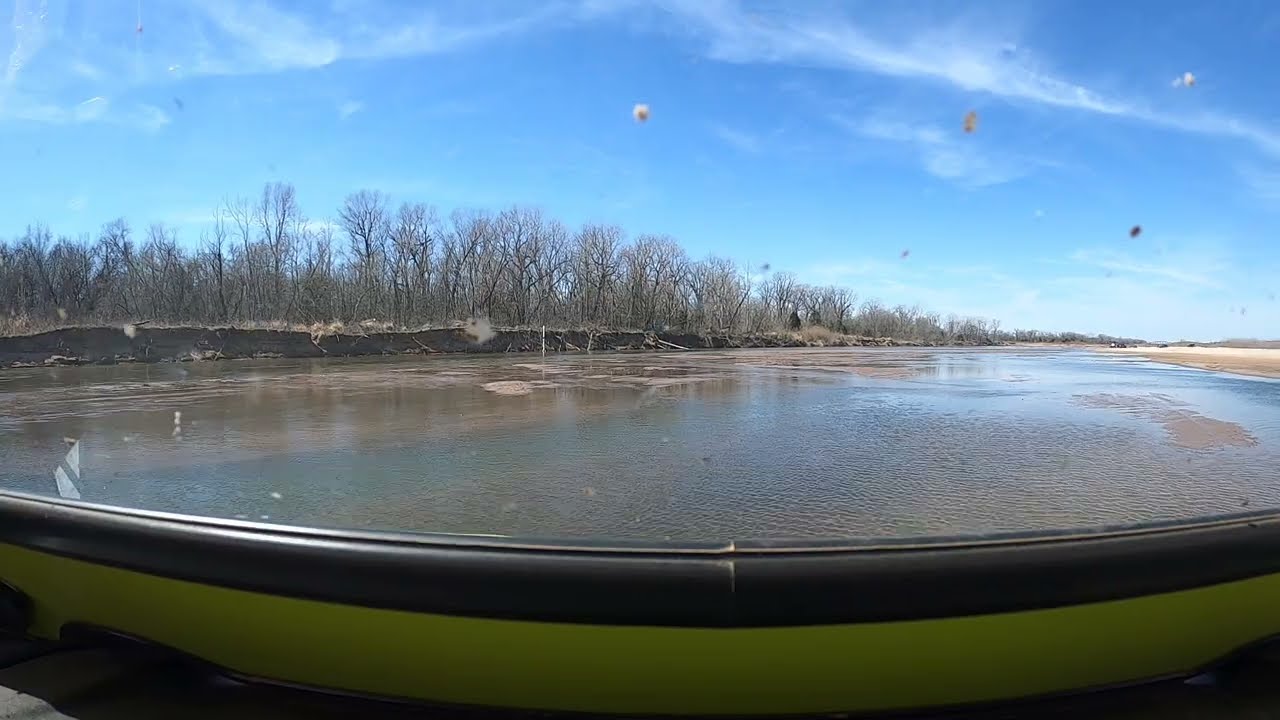The image depicts an outdoor scene viewed from the inside of a boat or raft, which features a green interior and a black edge. The viewpoint from the boat reveals a greenish-brown river with gentle ripples. On the left riverbank, a row of leafless trees lines the distance, standing on a berm of soil. In contrast, the right riverbank is characterized by a sandy area. The sky above is a bright blue, adorned with a few misty white clouds, adding depth to the picturesque setting. The waterway appears to be part of a natural landscape, possibly reinforced or shaped by man-made elements, as suggested by the structured berm.